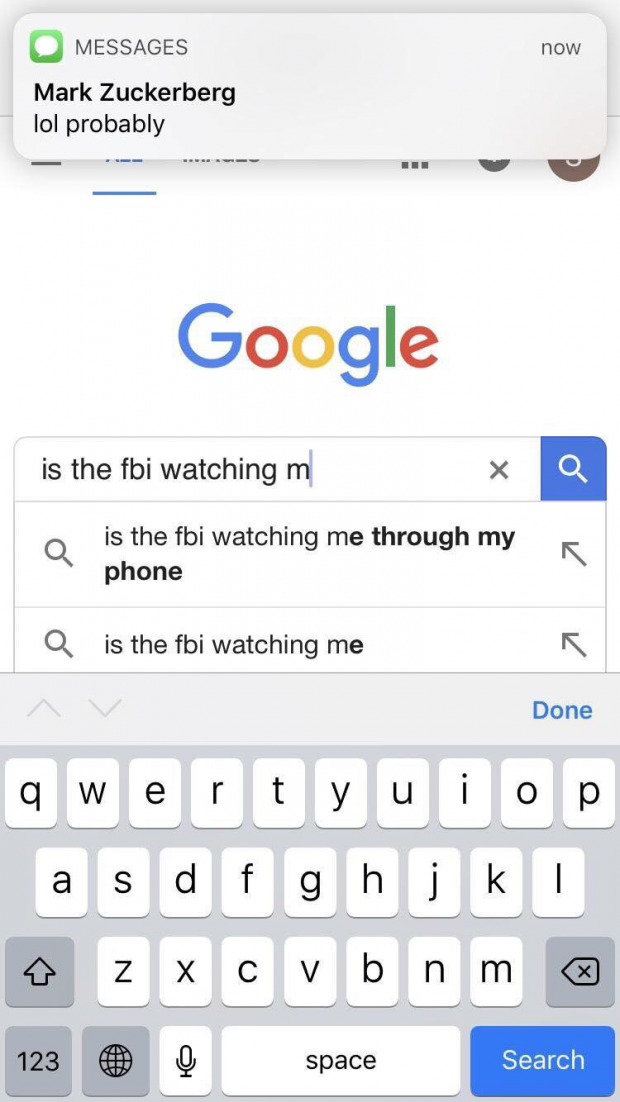The image depicts a Google search page where a person is typing queries. At the center of the screen, the word "Google" is prominently displayed in the characteristic Google colors: blue, red, gold, blue, green, and red. Below the logo, the gray outline of the search bar contains the query "is the FBI watching me", accompanied by a small gray 'X' and a white search icon against a blue background.

Under the search bar, predictive text suggestions appear. The first suggestion reads "is the FBI watching me through my phone" with a small arrow pointing up, followed by another suggestion, "is the FBI watching me", also with an arrow pointing up. 

The gray outline of an on-screen keyboard is visible, with white keys displaying black letters and numbers. Above the keyboard on the right, the word "Done" appears in blue. The keyboard includes a space bar, a voice input microphone icon, and a "123" key for switching to the numerical keypad. 

At the top of the screen, a banner notification is partially visible. It features a small green square with a white chat bubble icon indicating a message. The banner reads "Messages" in black, followed by "Mark Zuckerberg, LOL, probably" in darker black letters. This banner seems to have appeared due to the ongoing Google search.